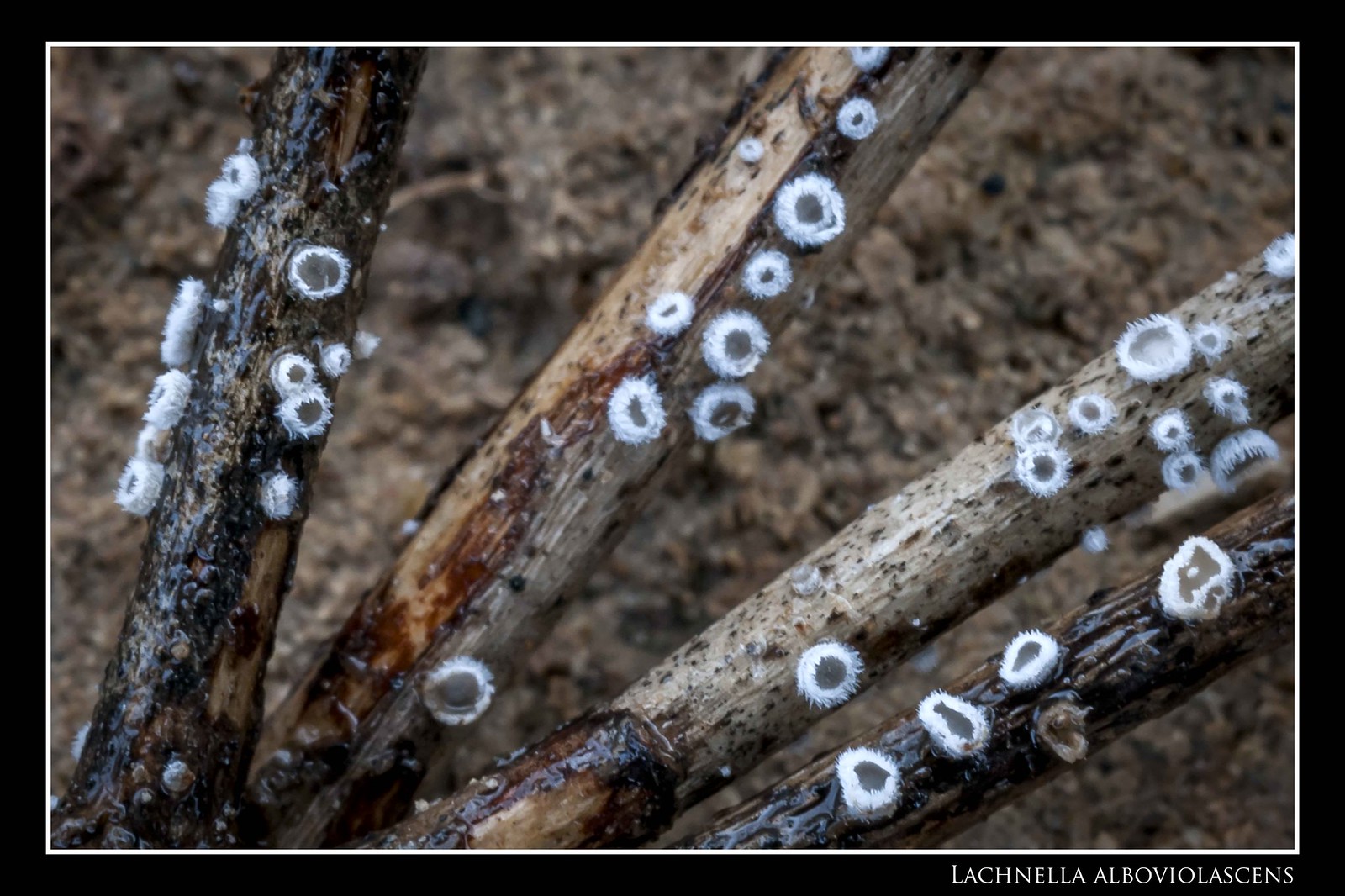This photograph, bordered by a prominent black frame with a thinner white inner frame, showcases the intricate details of several tree branches or sticks against a blurred forest floor backdrop of dirt and leaves. Central to the image are four distinct branches, each adorned with numerous small, circular fungi characterized by white edges and brown centers. The fungi, identified as Lachnella alboviolascens—spelled L-A-C-H-N-E-L-L-A A-L-B-O-V-I-O-L-A-S-C-E-N-S—are prominently featured throughout the length of each branch. This species’ technical name is elegantly displayed in white font in the bottom right corner of the photograph. The branches appear wet or shiny, possibly due to a substance covering them, further enriching the textural contrast within the image.